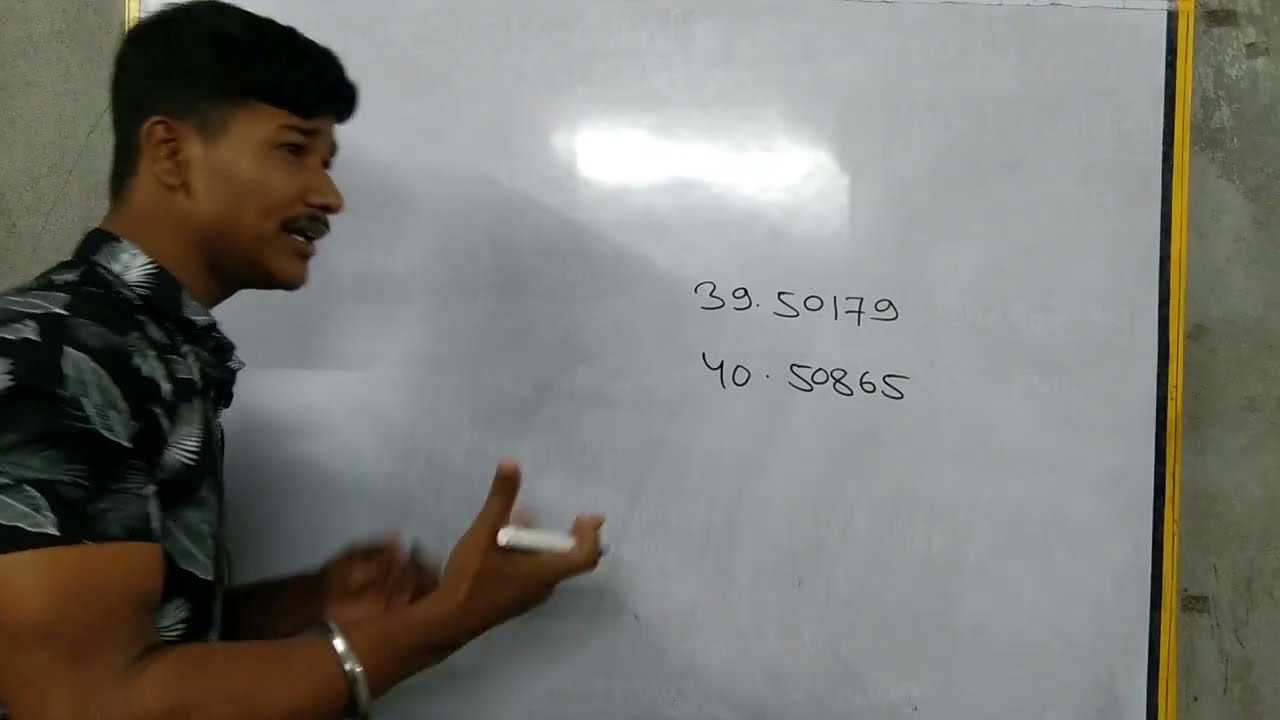The image captures a detailed side view of a man teaching in front of a whiteboard. The man, who has brown skin and dark hair, is dressed in a black short-sleeved collared shirt adorned with a white leaf design. He sports a mustache and a silver bracelet on his right wrist. His mouth is open mid-speech, and he is seen holding a white dry-erase marker, with motion blur suggesting he is gesturing with his hands. Behind him, the whiteboard, which has a yellow border, prominently displays the numbers "39.50179" and "40.50865" written in black. The board also reflects a light source, indicating a glare in the middle. The setting is against a gray wall where the whiteboard is mounted.